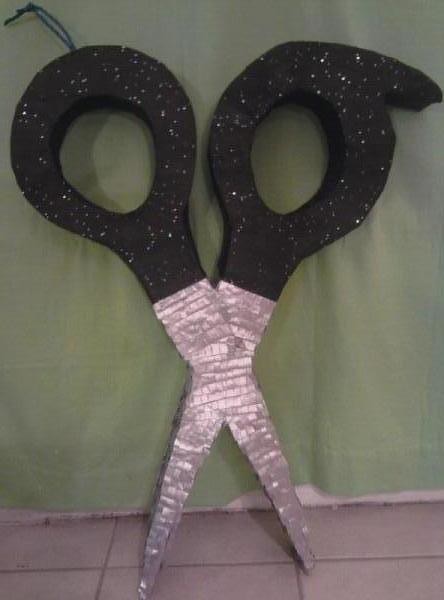The image features an oversized, intricately crafted pair of scissors. Leaning against a medium green curtain, the scissors stand prominently on a white and brown tiled floor. The handles, black with a speckling of glitter, add a touch of sparkle to the otherwise matte finish. The blades, constructed to mimic real scissors, are covered in a shimmering, silver material, likely tinfoil, enhancing their realistic appearance. The scissors are open wide, creating a striking visual. A string attached to the top left handle suggests that this handmade project, possibly a piñata, is designed to hang as a display piece. The overall composition showcases a detailed and creative arts and craft project, impressively simulating a large functional tool.